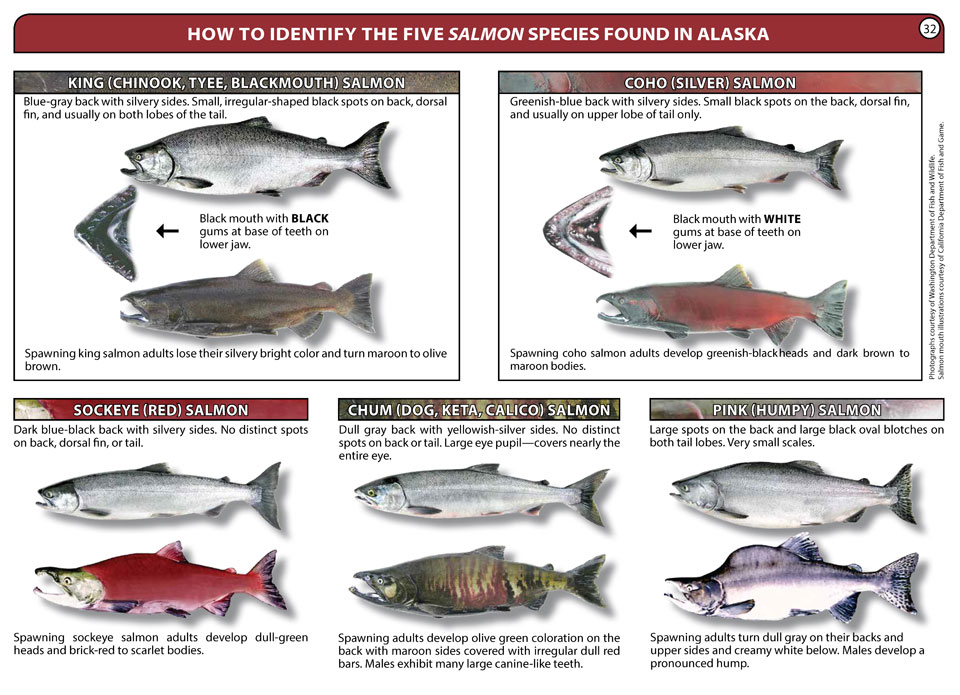This detailed poster, identified as poster number 32, is titled "How to Identify the Five Salmon Species Found in Alaska." The poster is divided into five sections, each dedicated to a different species of salmon: King (Chinook or Tyee or Blackmouth), Coho (Silver), Sockeye (Red), Chum (Dog or Keta or Calico), and Pink (Humpy). Each section features images and comprehensive descriptions of both the non-spawning and spawning phases of the fish.

The King Salmon images depict a silvery fish with a blue-gray to black back, characterized by small, irregularly shaped black spots on the back, dorsal fin, and usually on both lobes of the tail. The text notes that adult spawning King Salmon lose their bright silver color, turning blue to olive-brown, and are distinguished by black gums at the base of their teeth on the lower jaw.

Similarly, the other species are illustrated with descriptions of their distinctive features during both life phases. For instance, the Coho Salmon, also known as Silver Salmon, and Sockeye Salmon (Red) show significant changes in appearance from their non-spawning silver phases to their vibrant spawning colors. Chum Salmon, also called Dog, Keta or Calico, and Pink Salmon (Humpy) are also detailed, each with unique characteristics highlighted.

The sections are outlined in red or gray, with black writing detailing the specific identifying traits of each fish, helping readers distinguish between the species and understand how they change from non-spawning to spawning phases. This informative and visually rich poster provides an extensive guide for identifying the five major salmon species found in Alaska.